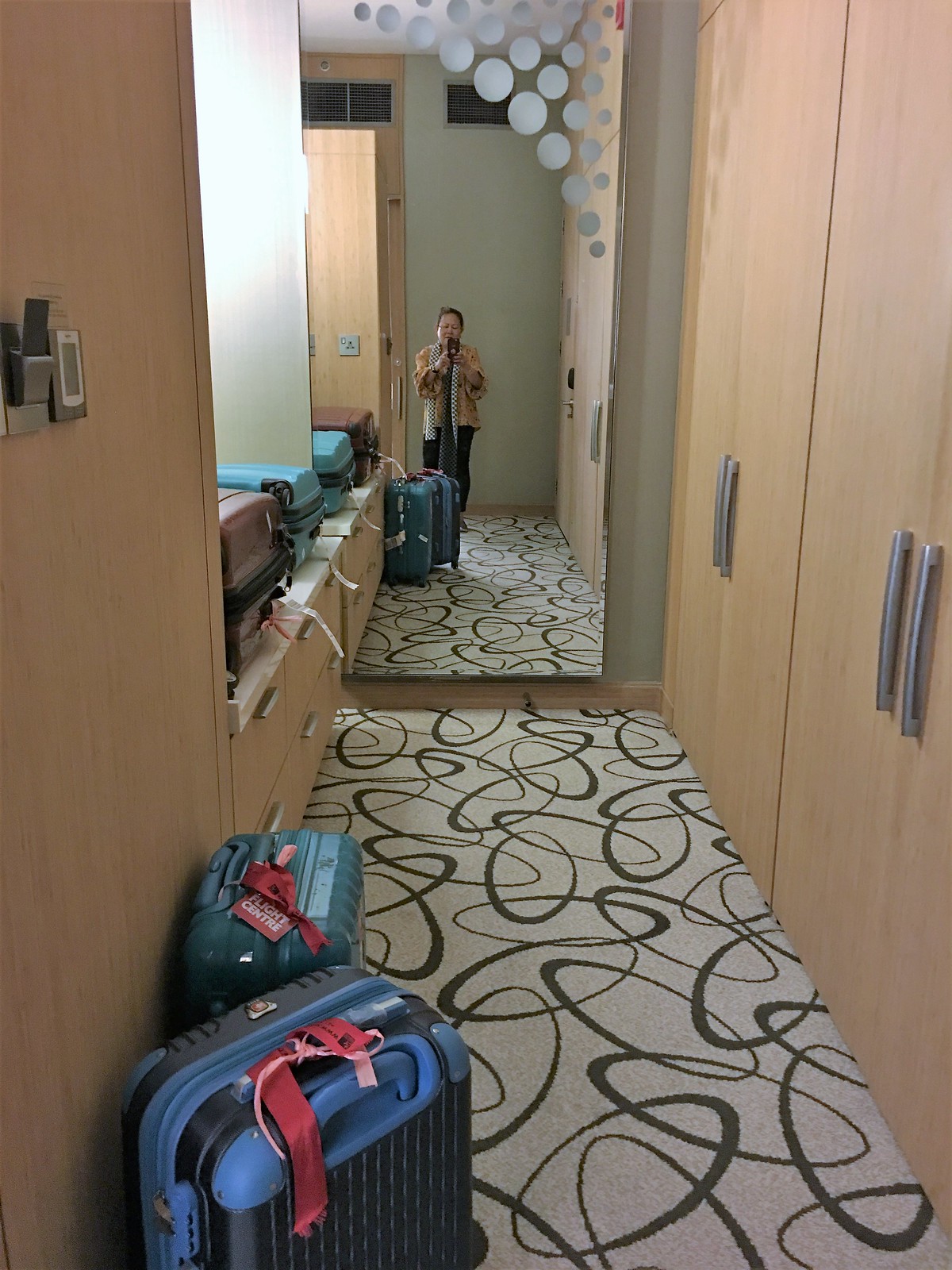The image captures the scene of a hallway, likely within a hotel or cruise ship. The setting boasts a detailed and intricate carpet design featuring beige and cream tones with intersecting olive or gray ovals. Lining the hallway are wooden cabinet doors, predominantly birch-colored, along with a heating system thermostat and a countertop with drawers on the left side.

A full-length mirror, adorned with bubble-like etched circles in the upper right corner, reflects an Asian woman taking a selfie. She is dressed in a brown jacket, black pants, and a loosely hanging black and white checkered scarf. In her hand is a phone, assisting in snapping the photograph. Scattered around are four suitcases: two on the ground in the foreground and two on the countertop on the left. The ground suitcases include a brown bag with blue trim and a green one, both tagged with red ribbons. On the counter, there are a brown suitcase and an aqua-colored one.